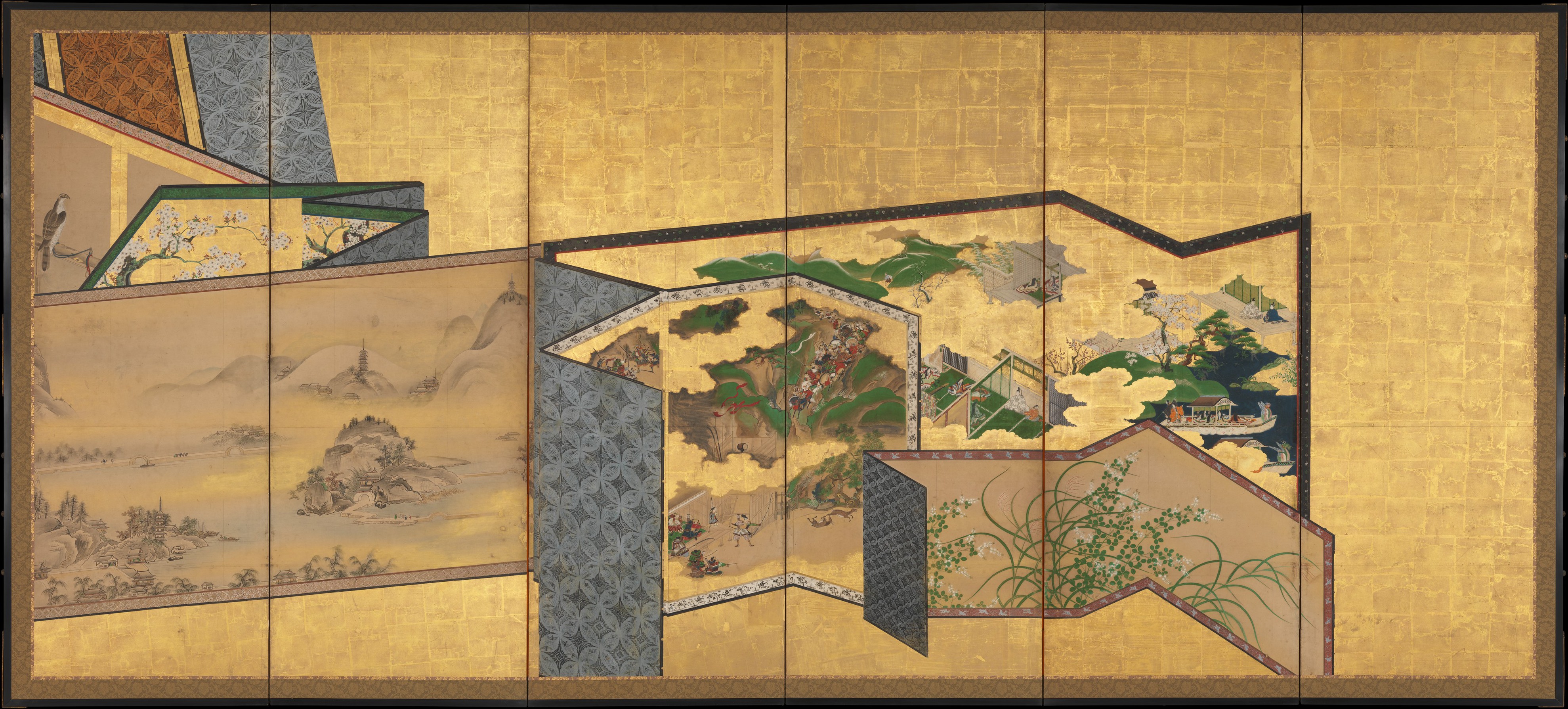This image captures an exquisite, horizontally elongated artwork, reminiscent of traditional Japanese art, structured into six distinct panels. The central theme of the canvas is a warm orangish-brown hue, bordered by a thin black line, creating a striking frame. Within each of the six main sections, there are intricate subsections resembling smaller, individual scrolls or paintings, giving the appearance of paintings within paintings or frames within frames.

These subsections, seven in total, depict various serene landscapes and natural elements. The bottom right contains the smallest painting, featuring simple grasses or plants with minimal background detail. Adjacent to it, a larger panel portrays fragmented village scenes, suggesting a narrative spread across different dimensions.

To the left, another folded section showcases a mountainous area, seamlessly blending with a more pastoral, hazy landscape with soft line work and subdued coloring. In the top left, though partially obscure, one can glimpse a tree branch adorned with delicate flowers. Dominating the center is a vivid green depiction of rolling mountains, while in the foreground of this, wispy green leaves enhance the scene, adding depth and texture.

This elaborate composition, with its interwoven themes and layered perspectives, evokes the feel of multiple room dividers or canvases folded and unfolded within a singular, cohesive artwork.